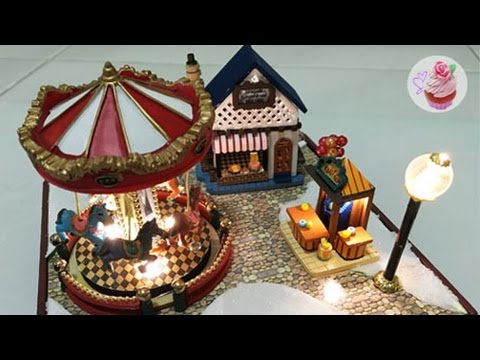The up-close photograph showcases a charming miniature village, intricately detailed with small ceramic dioramas. Central to the scene is a brightly lit merry-go-round adorned with red and white striped canopies and gold trim, its horses seemingly galloping across a checkered black and white floor. Adjacent to this whimsical carousel is an old-fashioned cottage with a market window, shaded by a red and white canopy, which displays various items for sale. Nearby, a small peaceful bench and table sit under a wooden canopy, softly illuminated by a hidden light, inviting someone to rest.

To the right, a quaint donut stand with a striped canopy and colorful balloons is visible, along with tables laden with delicious treats. The village is further brought to life with a black columned streetlight that provides ample lighting for the surroundings. Adding to the vibrant atmosphere, there is a display featuring a pink cupcake topped with green icing, pink flowers, and a rose, accompanied by a logo depicting a cupcake with two purple hearts. All these elements are set upon a cobblestone pathway, evoking the nostalgic feel of festive miniature villages often displayed during the holiday season.